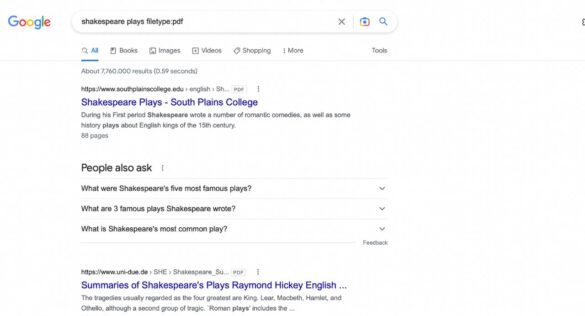This image appears to be a screenshot of a Google search results page. The search query entered is "Shakespeare plays file type: PDF." At the top, we see the familiar Google logo with the search bar displaying the search terms. Below the search bar, there's the navigational menu featuring options such as All, Books, Images, Videos, Shopping, and More. Adjacent to this menu is the Tools option, which is used to refine search results. The search yielded approximately 7,760,000 results in 59 seconds, as mentioned just beneath the navigational menu.

Just below this result summary, the first search result is displayed, featuring the web address leading to South Plains College. Following the link, a brief description regarding Shakespeare plays available at South Plains College is provided. Farther down the page, under this description, there are double spaces separating this section from the "People also ask" section, where related questions are listed to offer additional information that searchers might find useful.